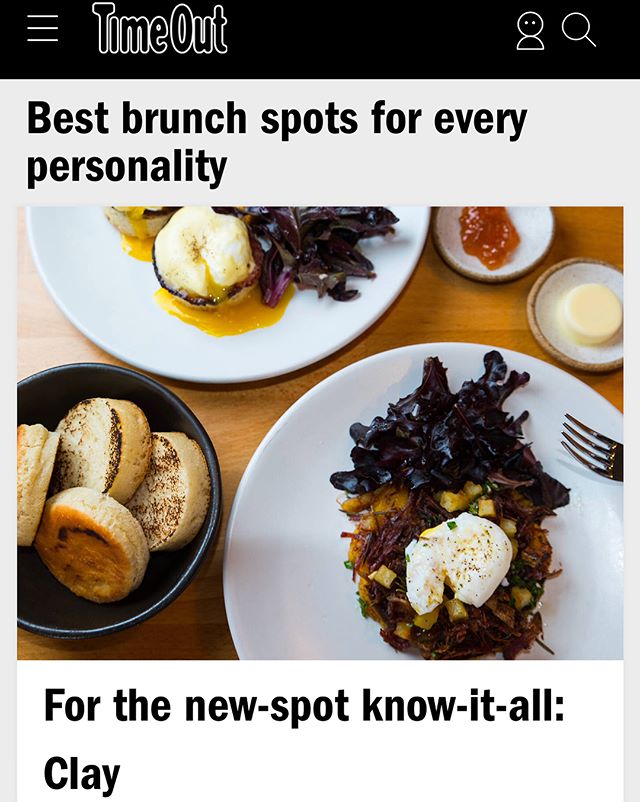The image features a simple, mock-up graphic with various elements. At the top, there's a black header bar containing a hamburger menu icon on the left and a profile graphic on the right, depicting a head and half a torso alongside a magnifying glass icon in a somewhat playful, outlined font. Below this header, a pinkish-grey field holds the text "Best brunch spots for every personality," followed by a subtitle at the bottom stating, "For the new dash spot know it all clay."

The main focus of the image is an overhead photograph of a brunch setting. Two large white plates are artfully angled, showcasing their contents. The top plate features what appears to be poached eggs atop a biscuit, with yolks flowing out, accented by a shiny red cabbage or cooked seaweed. The bottom plate mirrors this with a poached egg placed over shredded beef, accompanied by either chunks of potato or pineapple. Off to the left, a grey bowl contains several rolls or biscuits, and two small dishes hold what might be jelly and butter. A fork is seen partially entering the frame from the right, placed on the bottom plate. The entire setup exudes a casual yet appetizing brunch environment.